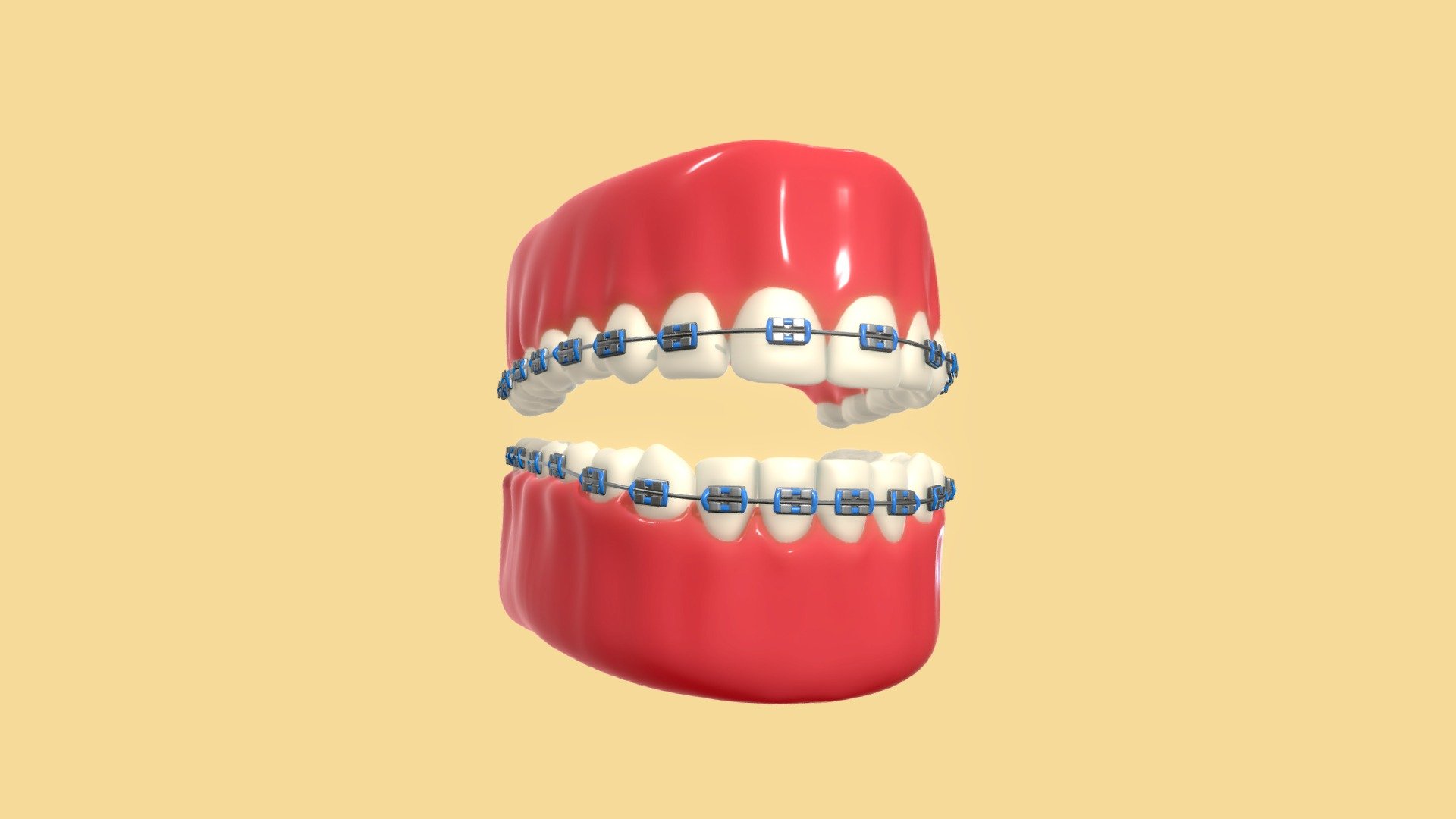The image depicts a highly detailed, computer-generated 3D model of a set of human teeth and gums, prominently showcasing braces. The background is a solid yellowish or pale beige color, creating a stark contrast with the dental model. The gums are a rosy red, appearing thick and glossy, giving a somewhat plastic look. Both the top and bottom rows of teeth are visible, slightly apart, revealing healthy, bright white, and well-aligned teeth. These teeth are fitted with traditional metal braces, which feature silver brackets and connecting wires. Each bracket includes a blue rubber band, contributing to the clinical detail of the model. The teeth and braces are symmetrically aligned, and the perspective of the image is slightly angled, offering a view of the back teeth on the top row. This illustrative model is likely designed for educational purposes, such as demonstrating how braces work in a dental setting.